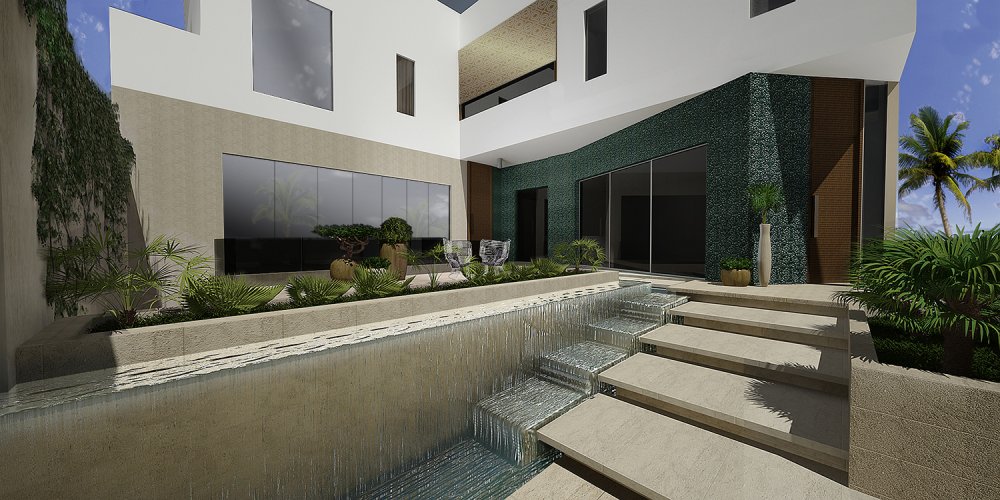The image captures the front of a very fancy-looking, modern minimalist two-story house or apartment building. The entrance is accentuated by a series of gradual beige-colored steps, about four or five, leading up to a front door. Adjacent to these steps, there's a small waterfall cascading down from a side wall, which also seems to nourish the smart garden sections lined with green shrubbery and plants, including palms and vines. The house has an architectural design featuring numerous large, tinted, sun-protected windows that provide ample natural light. The structure extends to both the left and right, with the main part of the building showcasing a sleek combination of white, gray, and dark green sections. Notably, the entryway is adorned with dark blue tiles, and the second story includes a mix of large and smaller rectangular windows, one of which has golden-colored blinds. Adding to the scene, the background suggests a tropical locale with blue skies, scattered clouds, and some palm trees.